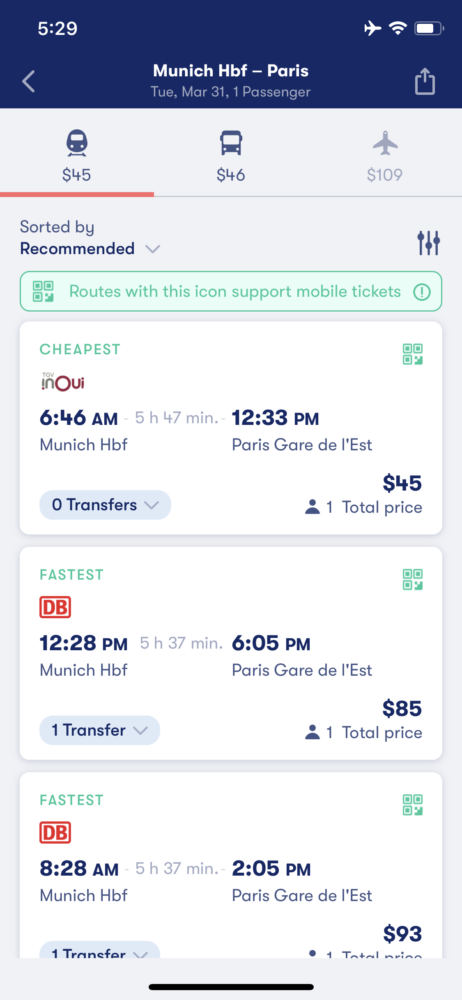The image displays the screen of a mobile device. In the upper left corner, the time is shown as 5:29 in white text. The upper right corner features three icons: the first for airplane mode, the second for Wi-Fi, and the third for battery life. These icons reside on a blue horizontal bar at the top of the screen.

Beneath this bar, the screen displays several transportation options with associated costs. The train icon, highlighted and underlined in orange, shows a fare of $45. The bus icon next to it lists a fare of $46. Additionally, there is a greyed-out airplane icon marked with a fare of $109.

The lower portion of the screen details three different train routes. The topmost route is labeled "Cheapest" in green text. This section conveys various route options, organized to assist the user in making travel decisions.